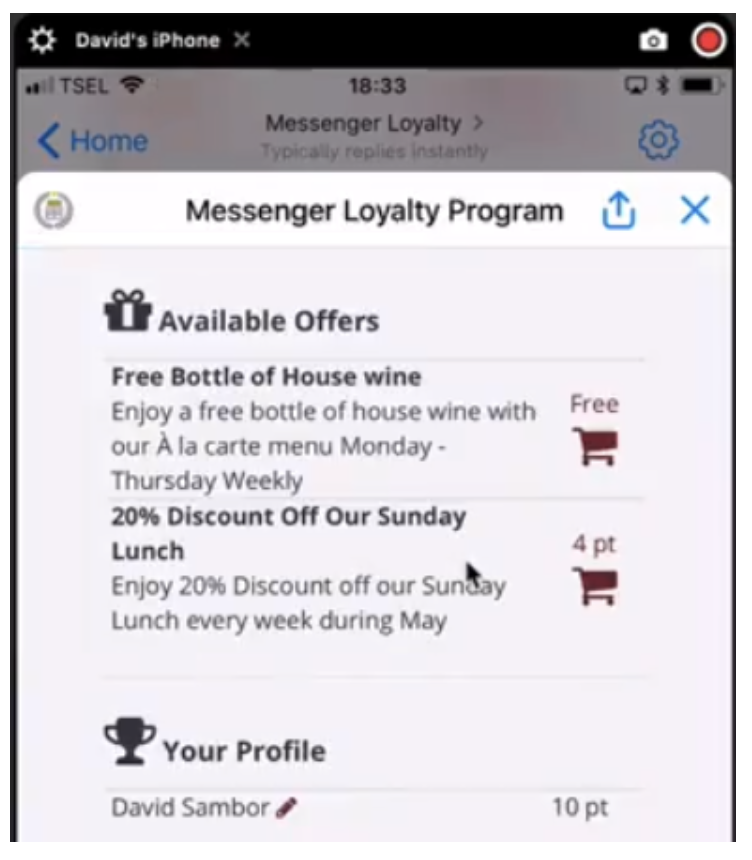Captured on the screen of David's iPhone, this image provides a detailed view of a loyalty program interface within a messaging app. The top part of the screen is bordered by a black rectangle, displaying "David's iPhone" flanked by a gear icon on the left and a close icon (X) on the right. On the top right corner, there is an evident red button resembling a recording indicator encircled in white.

Just below the header, a blue text labeled "Home" is positioned next to a left-pointing arrow. Further down, the text "Messenger Loyalty" alongside "Messenger Loyalty Program" is clearly visible. Accompanying this text is a black and white icon designed with leaves.

Progressing downward, a blue "Upload" button and another close icon (X) can be found. Below these, a cartoonish gift icon introduces the "Available Offers" section, where a highlighted deal reads "Free bottle of house wine." The offer details include “Enjoy a free bottle of house wine with our a la carte menu Monday through Thursday weekly” next to a grocery cart icon marked "Free." 

Additionally, there is a 20% discount offer noted below, followed by the user's profile information. Displaying "David Sabur" and a point tally, the profile reveals that David currently has 10 points accumulated in the loyalty program.